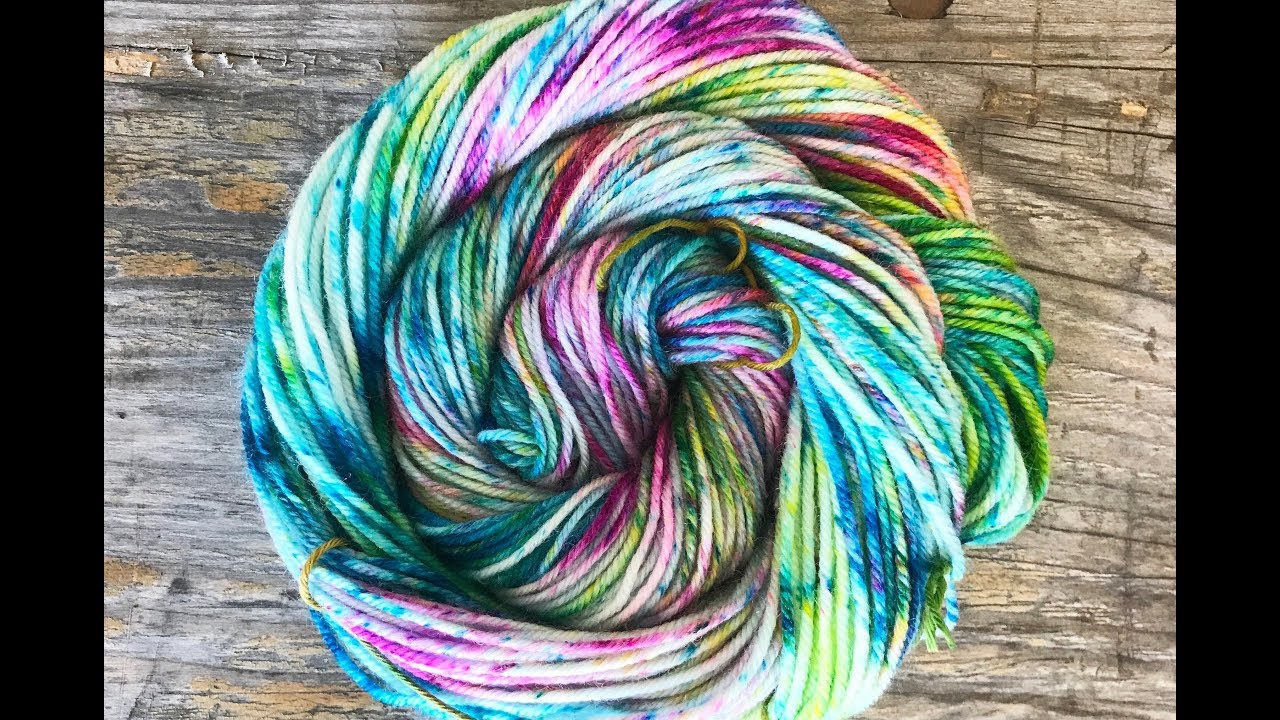The image showcases a tightly bundled cluster of yarn, arranged in a spiral pattern from a top-down perspective. The yarn, which is fairly thin, displays a vibrant array of colors including pink, white, blue, green, yellow, red, purple, lavender, and orange, creating a rainbow-like cornucopia. This cluster is centered in the photograph, exhibiting a circular formation where the yarn wraps around itself multiple times, forming concentric circles that taper inward to the very center. The yarn rests upon a wooden table or work surface, which is characterized by its rough, unfinished texture and visible gouges, lending a rustic, well-used appearance. Framing the image are two vertical black lines positioned at the farthest right and left edges. The overall composition accentuates the colorful, swirling yarn set against the contrasting ruggedness of the wooden table.